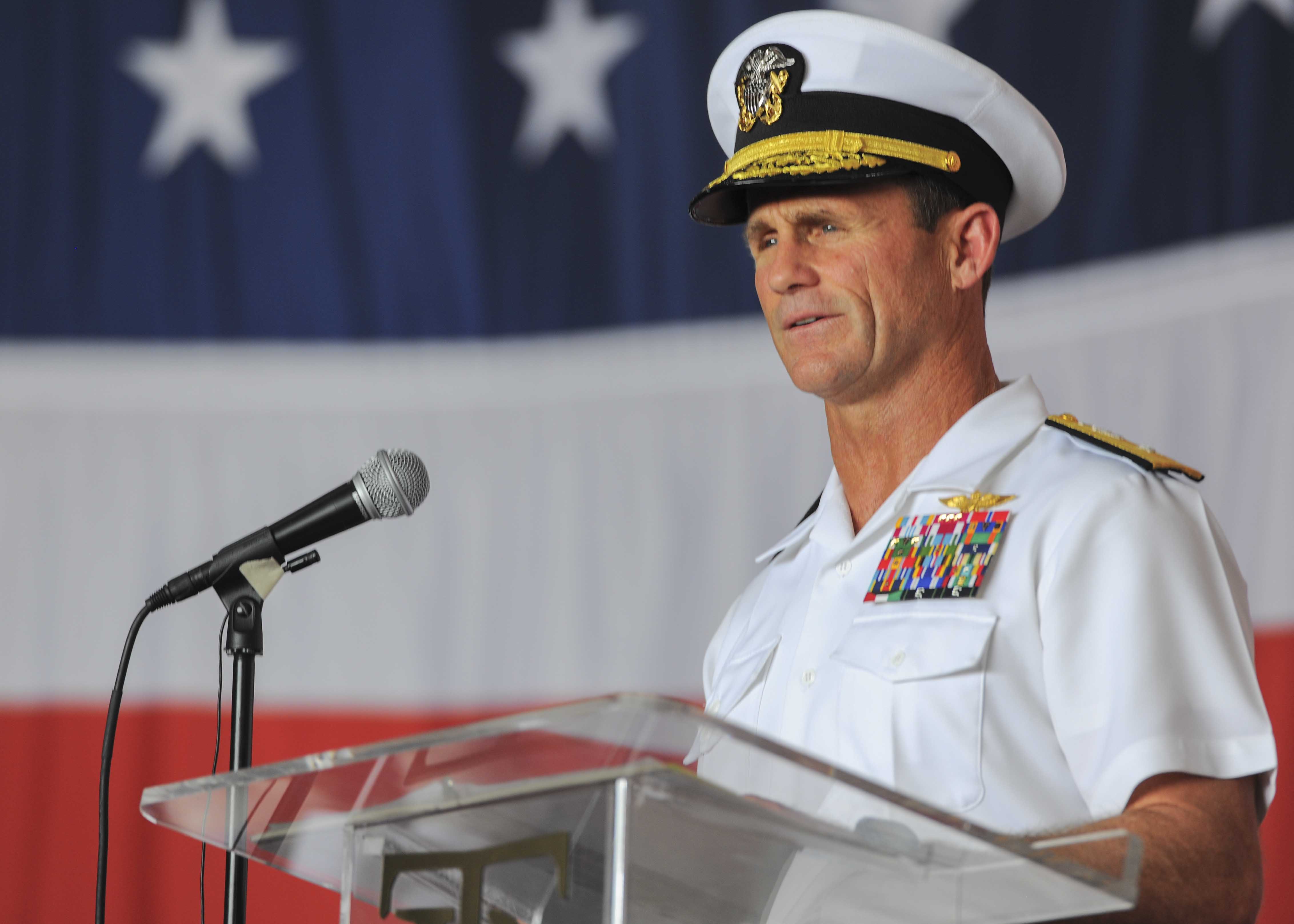In the image, an older Caucasian naval officer, likely between 50 and 60 years old, stands at a clear glass podium fitted with a black microphone. He is donned in a pristine white military uniform complete with a short-sleeved coat, featuring two front pockets and epaulettes with gold trim on the shoulders. His white hat, adorned with a black brim and gold stripe, prominently displays a large insignia at the front. On his left upper chest, a rectangular array of colorful medals and ribbon pips is showcased above his breast pocket. The officer appears composed, gazing toward the left without any discernible emotion. Behind him, a blurred United States flag with blue, white, and red stripes and white stars on the blue field marks the backdrop, along with a large indistinct banner featuring similar patriotic colors. The podium in front of him also holds a piece of paper, hinting that he is likely delivering a prepared speech.